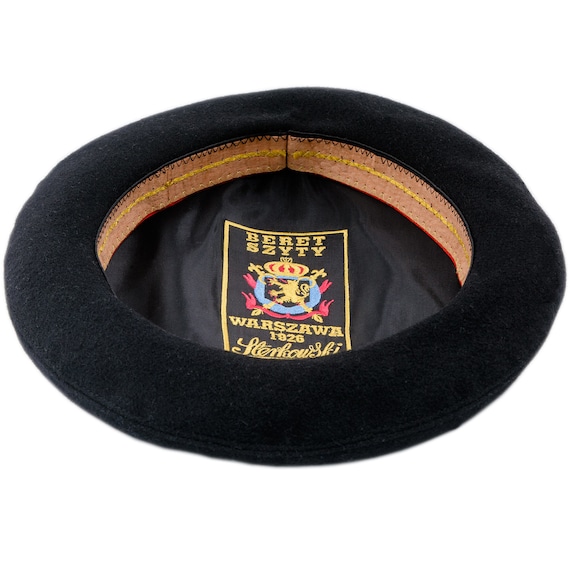The image depicts an inverted black beret, emphasizing its interior. The beret appears to be made of high-quality black felt and features a light tan leather band stitched with yellow and black thread around the rim. At the center of the interior, there's a detailed black and gold patch in Polish, showcasing a regal crest with a gold lion on a shield, topped by a golden crown and adorned with embellishments. Beneath the crest, a red banner displays the word "Beret," followed by "S-Z-Y-T-Y" and "Warzawa 1926." The word "Stankowski" is written in cursive below this information, though it is partially obscured. The intricate design includes fleur-de-lis and what appear to be pink banners whose ends resemble human hands making an "I love you" sign.